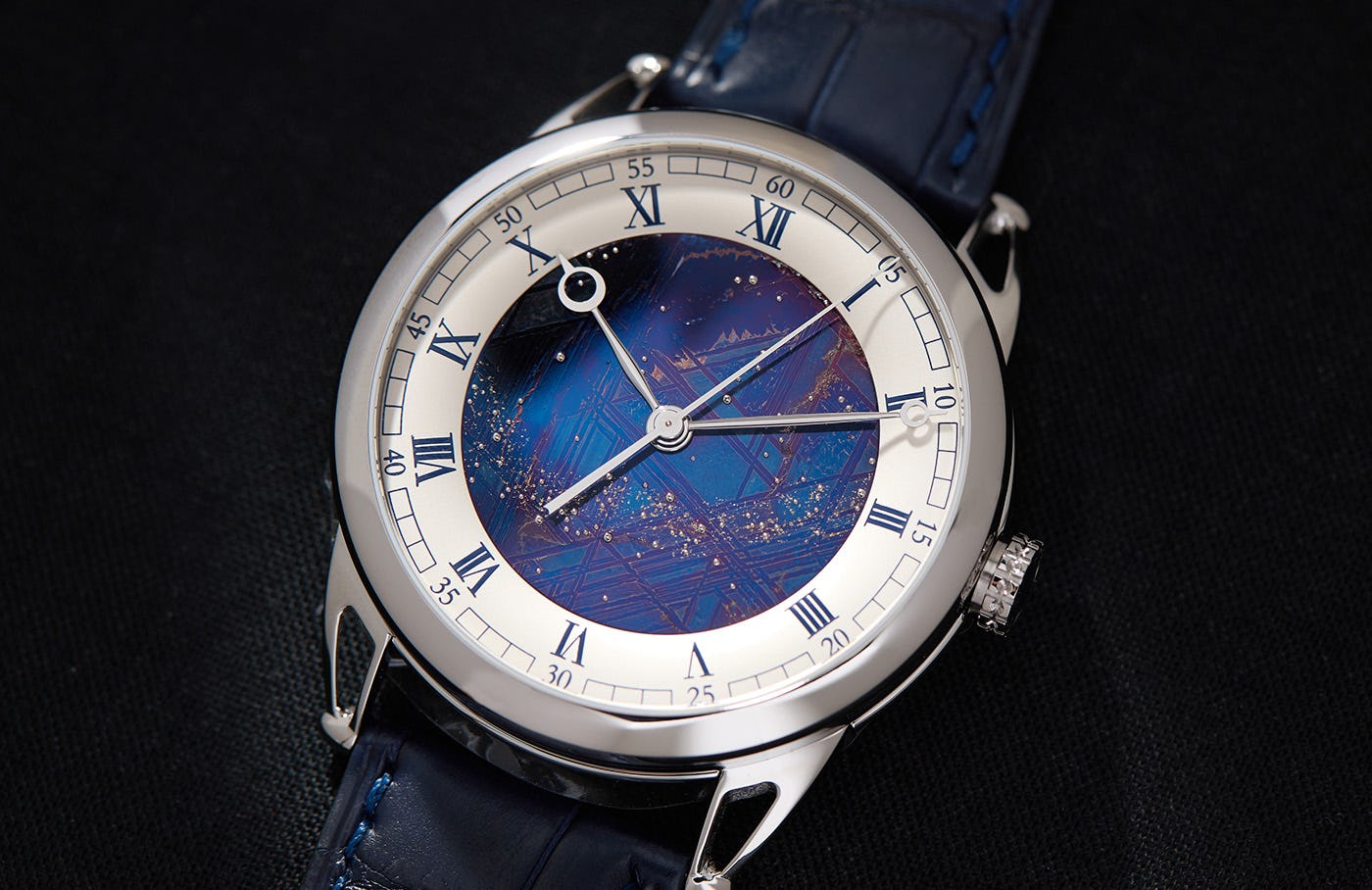This detailed image features a sophisticated wristwatch on a black background, slightly diagonal to the left. The watch boasts a dark blue leather strap, stitched with lighter blue threads. The polished silver hardware complements the refined aesthetic. The watch face is encased in a silver rim with a white interior and Roman numerals marking the hours. Surrounding the Roman numerals, there is a secondary scale for tracking seconds, marked in increments of 5 from 0 to 60.

The centerpiece of the watch is an intricate blue circle, reminiscent of a motherboard circuit, adorned with geometric triangle shapes in purple and glittery golden specks akin to stars. This evokes a celestial scene. The hour and minute hands are silver with circular ends and pointed tips, while the second hand features a distinct circle with a tiny beak-like point at the end.

The watch's decorative dial, used for adjusting time, is offset with what appears to be diamond embellishments, accentuating its luxury. The current time displayed is approximately 10:10.